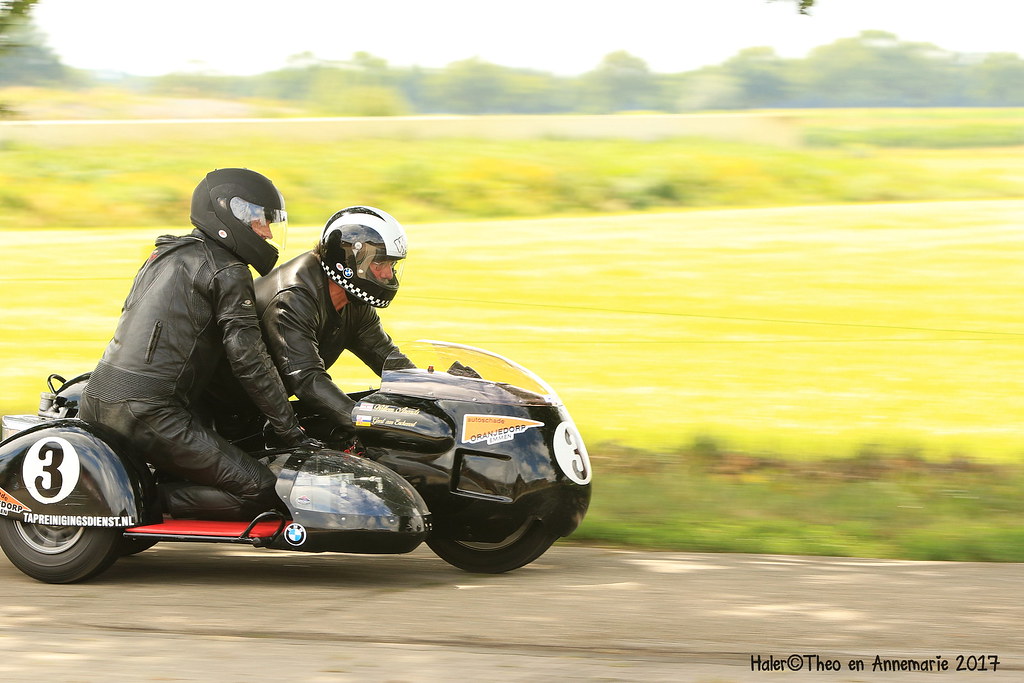The image captures an exhilarating high-speed motorcycle race featuring a two-man team on a sleek, black racing bike equipped with a sidecar. The motorcycle, bearing a distinct BMW logo and the number three prominently displayed in black on white circles at the front and on the sidecar's rear wheel, showcases its aerodynamic design and low profile. The riders are clad in full protective gear, with the driver wearing a leather jacket and a black-and-white helmet, and the sidecar passenger in leather coveralls and a matte black helmet. The dynamic action of the race is evident as they navigate a shaded corner with the blurred background, indicative of their breakneck pace. The scene is set on a brown, hard surface track bordered by a lush green field that transitions into yellow grass and trees in the distance. The photograph, taken on a sunny day, exudes a sense of speed and precision as the focused passenger leans to aid in the motorcycle’s rapid maneuvering. The image also includes a subtle copyright note at the lower right, reading "HALER, H-A-L-E-R, copyright Theo N. N. Marie, 2017."